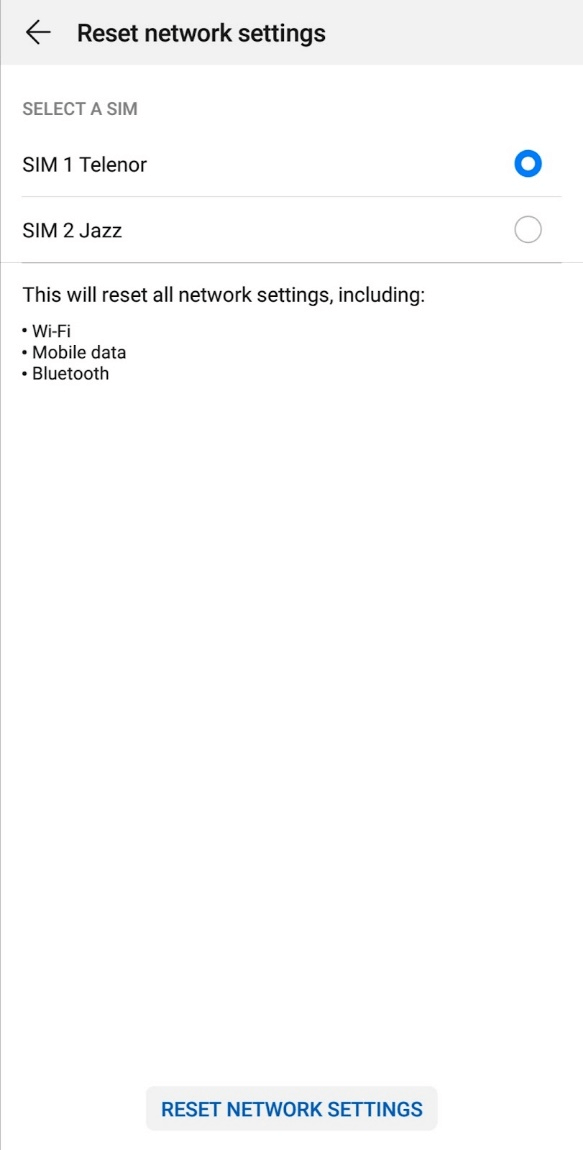The image depicts a smartphone settings page titled "Reset Network Settings." At the top, there is a black back arrow on a gray bar. The main header "Reset network settings" is displayed in black text. Below it, users are prompted to "Select a SIM" with two options: "SIM 1: Telenor" and "SIM 2: Jazz." "SIM 1: Telenor" is currently selected, indicated by a blue circle next to it. The accompanying text explains that initiating a reset will revert all network settings, including Wi-Fi, mobile data, and Bluetooth, to their default configurations. The page mostly uses a white background with black and gray text, providing a simple and clean interface. At the bottom of the screen, there is a prominent blue button labeled "Reset network settings." This page is typical of the network settings section found on most smartphones.